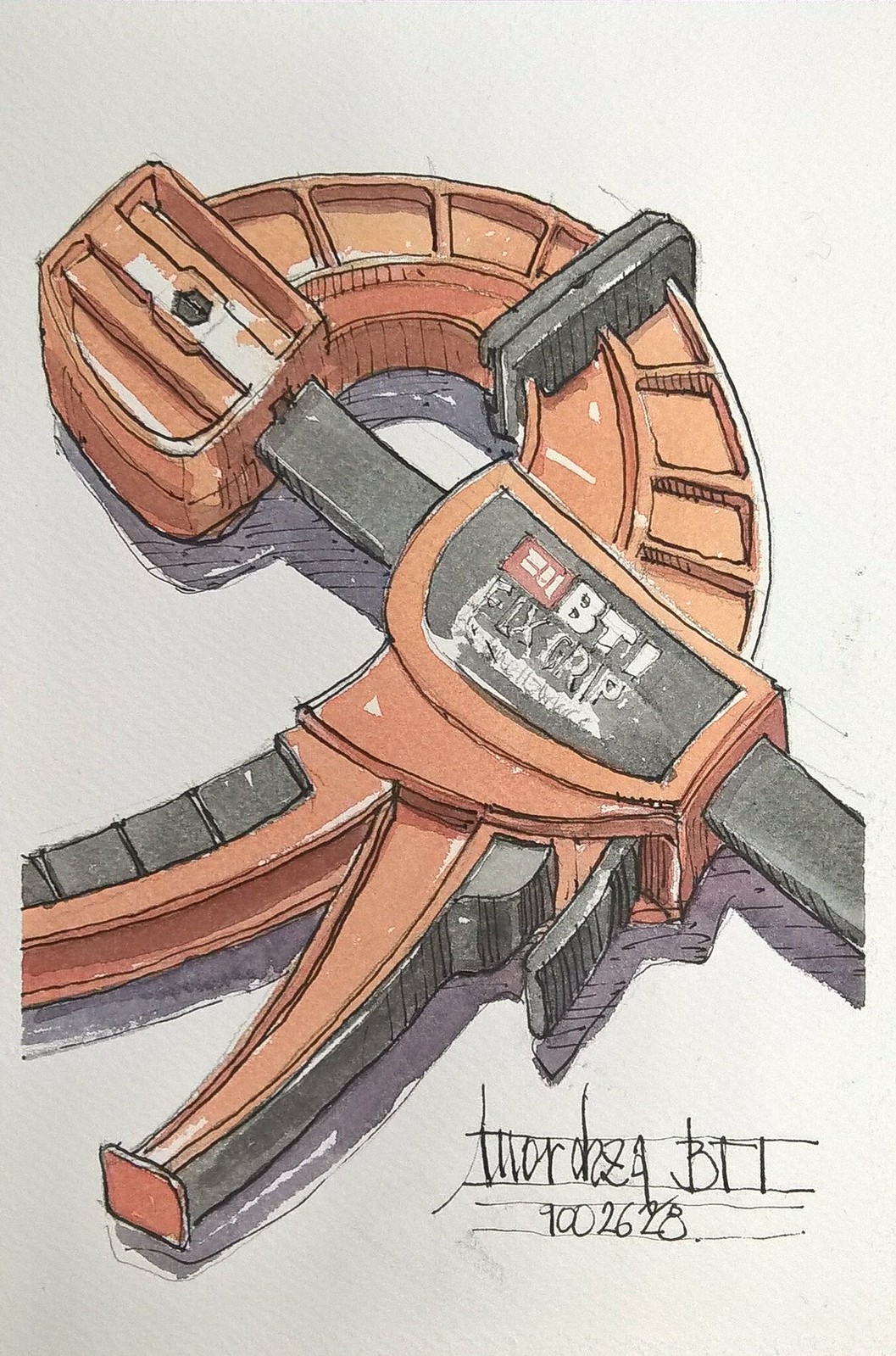The image is a detailed artist rendering, created using pen and ink and enhanced with watercolor paints, depicting a tool labeled "BTI Fix Grip." The artwork, which appears on a white background, is done in shades of brown, gray, and orange. The BTI Fix Grip is oriented slightly angled towards the upper right, showcasing its curved top resembling a comma shape. The handle, extending from the bottom right, is flat and square at the end, suggesting it might push out something like staples. Notably, it includes a small black lever under the curved section. The tool's logo, "BTI Fix Grip," is prominently displayed, with additional numbers, possibly "211," inscribed on the top. The artist's signature and the date "9002628" are written in a lined space in the bottom right corner, mimicking a piece of lined paper. The overall rendering maintains a mysterious, tool-like aesthetic.